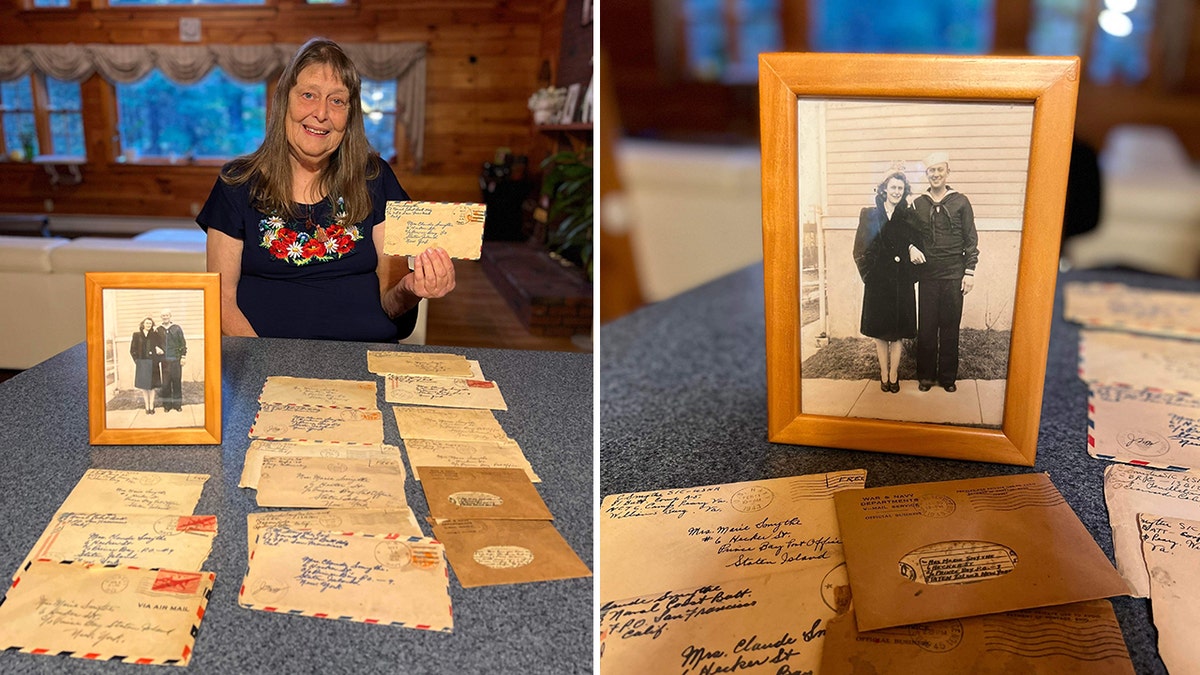The image consists of two vertical rectangles placed side by side, separated by a thin white line. The left side captures an older woman, likely in her 60s, sitting at a countertop with a cabin-like wooden window in the background. She has long brown hair cascading over her shoulders, wears a black short-sleeve floral patterned shirt, and is smiling gently. The countertop is black and gray speckled with very fine dots, and scattered across it are multiple old, light tan envelopes with blue ink and red, white, and blue dashes along the edges, suggesting they are from the World War II era. The woman is holding one such envelope. Also on the counter are three more envelopes in front of a small, 5x7 wooden picture frame containing a black and white photo of a man in a Navy uniform and a woman in a long black dress or coat, believed to be her parents, Marie and Claude Smythe. The right side of the image provides a close-up of this framed photograph, further highlighting the details of the Navy uniform, the sepia tone of the picture, and the wooden frame. Additional envelopes are scattered near the picture, further emphasizing their historical significance.